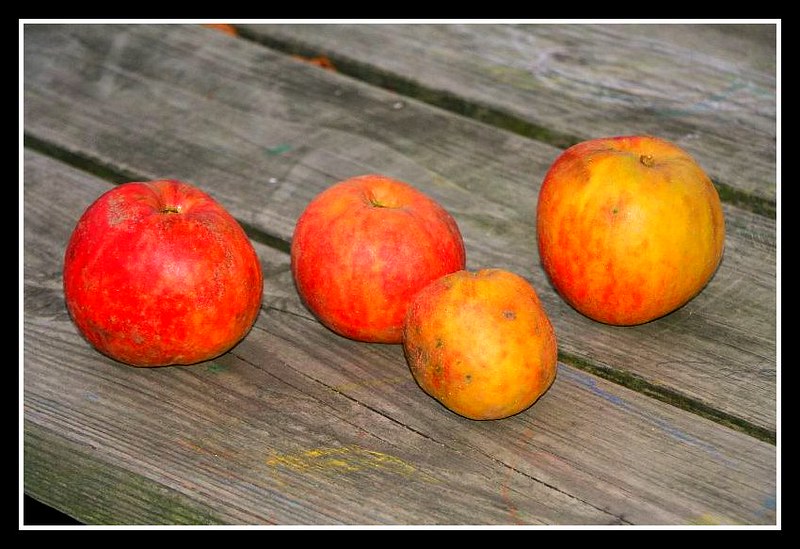The image showcases an aged, weathered picnic table, identifiable by its wooden slats and distinct spaces between them. The table, which might have been used for painting given its streaks of yellow, blue, and red, sits outside, with visible grass underneath. Atop the table are four pieces of fruit, predominantly red and orange, likely either apples, oranges, or peaches. They appear weathered and imperfect, with visible bruising, scaly skin, and small brown, pitted areas suggesting age or minor damage. One fruit, notably orange, shows significant bruising, while another smaller one in the front has a noticeable moldy appearance. The rest look more intact but still display signs of age. These fruits are arranged in a way that suggests they might be sitting on their stems, emphasizing their wear and weathering as the central focus of the photo. The image has a black and white border, making the vibrant but aged fruits stand out starkly against the rustic backdrop of the old picnic table.